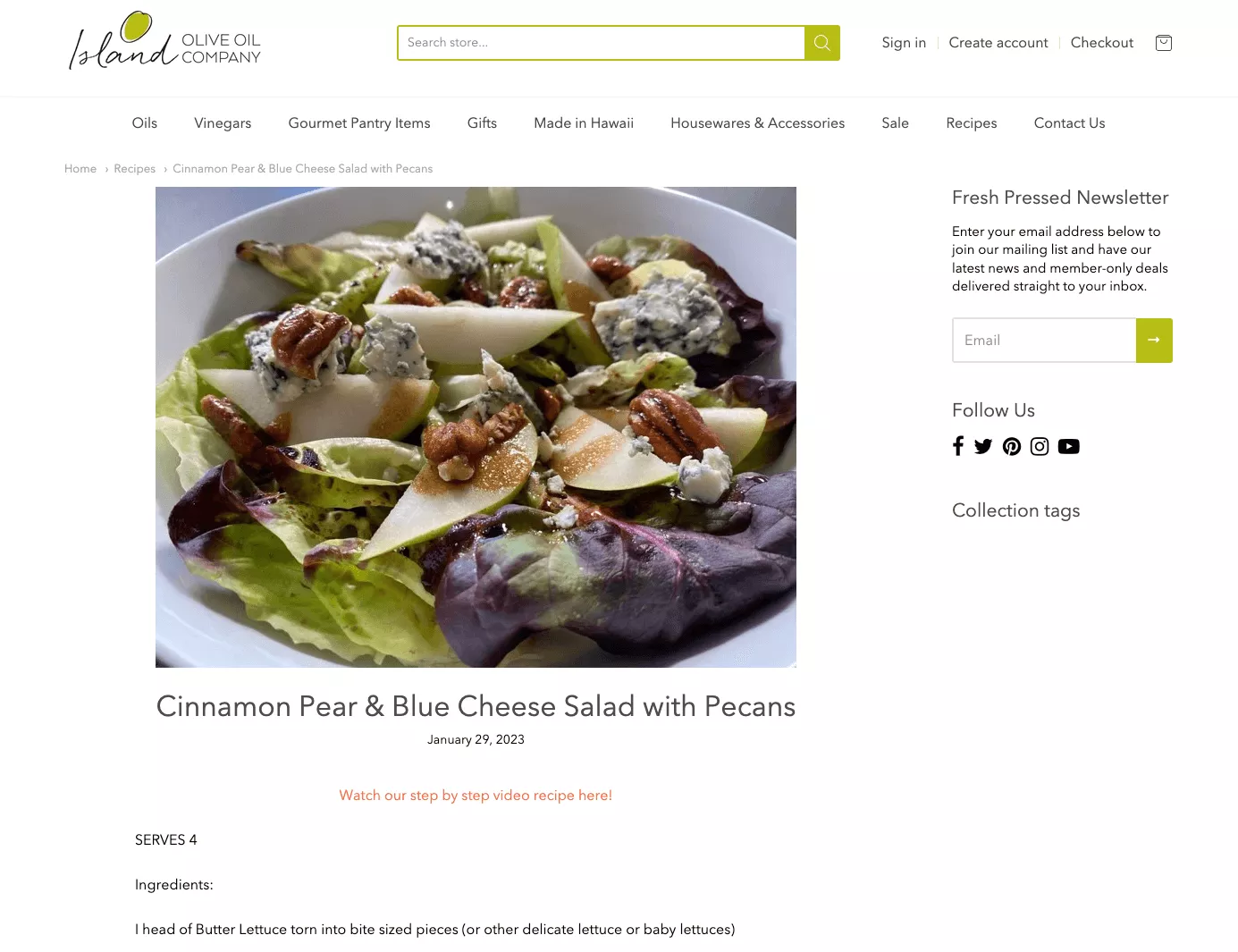This image is a screenshot of a website featuring a gourmet olive oil company. In the top left-hand corner, the website logo reads "Island" in elegant cursive script followed by "OLIVE OIL COMPANY" in bold capital letters. At the center of the top navigation bar, there is a search bar flanked by several buttons on its right: "Sign In," "Create Account," "Checkout," and what appears to be a calendar icon.

Beneath this top bar is a gray dividing line, followed by a secondary navigation menu that offers categories including Oils, Vinegars, Gourmet Pantry Items, Gifts, Made in Hawaii, Housewares and Accessories, Sale, Recipes, and Contact Us. 

The main content below this displays a vibrant image of a salad. The salad features lettuce, what appears to be butter lettuce, apple slices, pecans, and blue cheese. However, they are actually pears, not apples, which is confirmed by the caption below the image: "Cinnamon Pear and Blue Cheese Salad with Pecans." Beneath this caption, a red text states, "Watch our step-by-step video recipe here."

Starting the recipe, the text indicates:
- Serves four.
- Ingredients: One head of butter lettuce, torn into bite-sized pieces, or other delicate lettuce or baby lettuces.

To the right of the salad image, there's a segment inviting visitors to subscribe to the "Fresh-Pressed Newsletter." It prompts users to "Enter your email address below to join our mailing list and have our latest news and members-only deals delivered straight to your inbox." Below this prompt is a text box for email input, accompanied by an arrow pointing to the right.

The website also encourages social media engagement, featuring icons for Facebook, Twitter, Pinterest, Instagram, and YouTube under the "Follow Us" section.